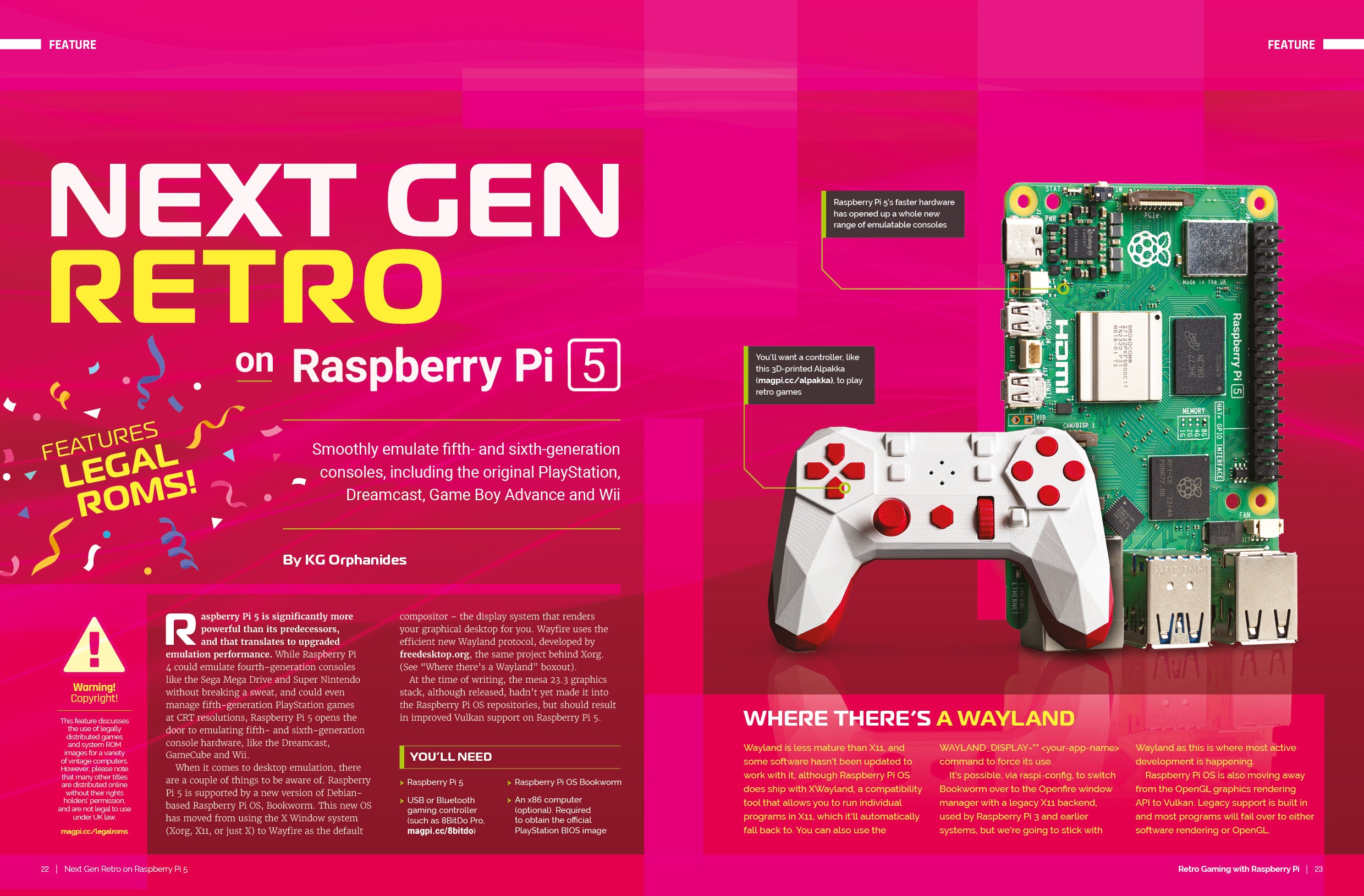The image depicts a vibrant two-page magazine spread titled "Next Gen Retro on Raspberry Pi 5" against a backdrop of deep pink hues, transitioning from light to dark. The left page serves as the article's introduction, with "Next Gen" in bold white letters and "Retro" in striking yellow, and underneath, "On Raspberry Pi" in white. The number "5" is enclosed in a white square beside the title. Prominent diagonally written yellow text states "Features Legal ROMs." The main body of the article, written in smaller white text, elaborates on the Raspberry Pi 5's capabilities to smoothly emulate fifth and sixth-generation consoles, including the original PlayStation, Dreamcast, Game Boy Advance, and Wii. 

The right page prominently displays a large image of the Raspberry Pi 5 circuit board, showcasing its intricate electronics. Adjacent to it is a sleek, white, angular game controller with red buttons, hinting at the device’s gaming applications. The red section at the bottom comprises additional text details, likely expanding on how to set up and utilize the Raspberry Pi for retro gaming. Overall, the spread is an eye-catching blend of visual and textual elements aimed at capturing the essence of modern retro gaming through Raspberry Pi 5.